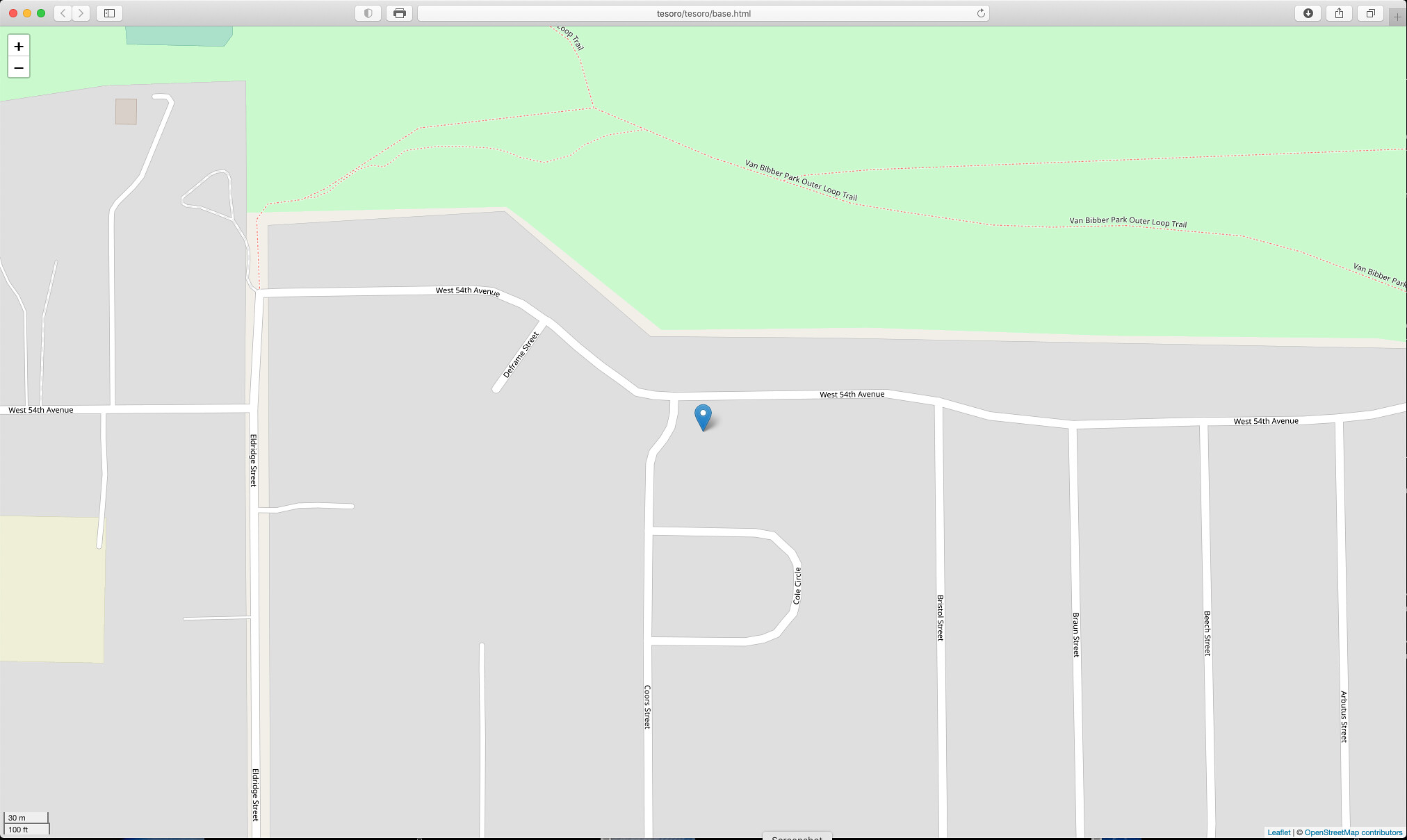This screenshot captures a map displayed on a Mac computer screen, identified by the distinctive red, yellow, and green window controls in the upper left-hand corner. The map, primarily rendered in shades of gray, white, black, and green, highlights a residential area. At the center of the screen, a blue indicator marks a specific location, seemingly at the intersection of two streets. The upper portion of the map features a green area, suggesting the presence of a park, golf course, or similar natural space. Street names are visible, providing detailed context to the viewer.